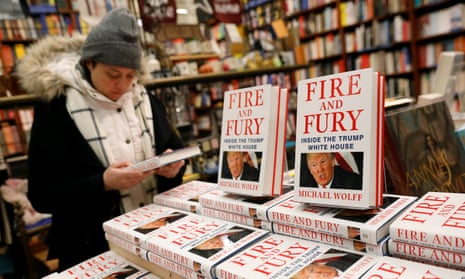This photograph captures a bustling bookstore scene with an extensive display of Michael Wolff's book, *Fire and Fury: Inside the Trump White House*. The table in the foreground is dominated by at least nine stacks of the book laid flat, with two rows of books propped up vertically for easy viewing. The cover of the book, which is prominently white with red text for the title and author's name, features an image of an irate Donald Trump with a blurred American flag in the background. 

A woman stands to the left of the display, engrossed in reading the back cover. She is dressed warmly in a winter coat that is black with a fur-lined hood, a gray beanie cap, a white underneath layer, and a black and white scarf. The setting appears to be a large bookstore, potentially in a high-traffic area like a train station or airport, given its commercial ambiance. The background is filled with more books on shelves, blurred to enhance the focus on the woman and the *Fire and Fury* display in the foreground.